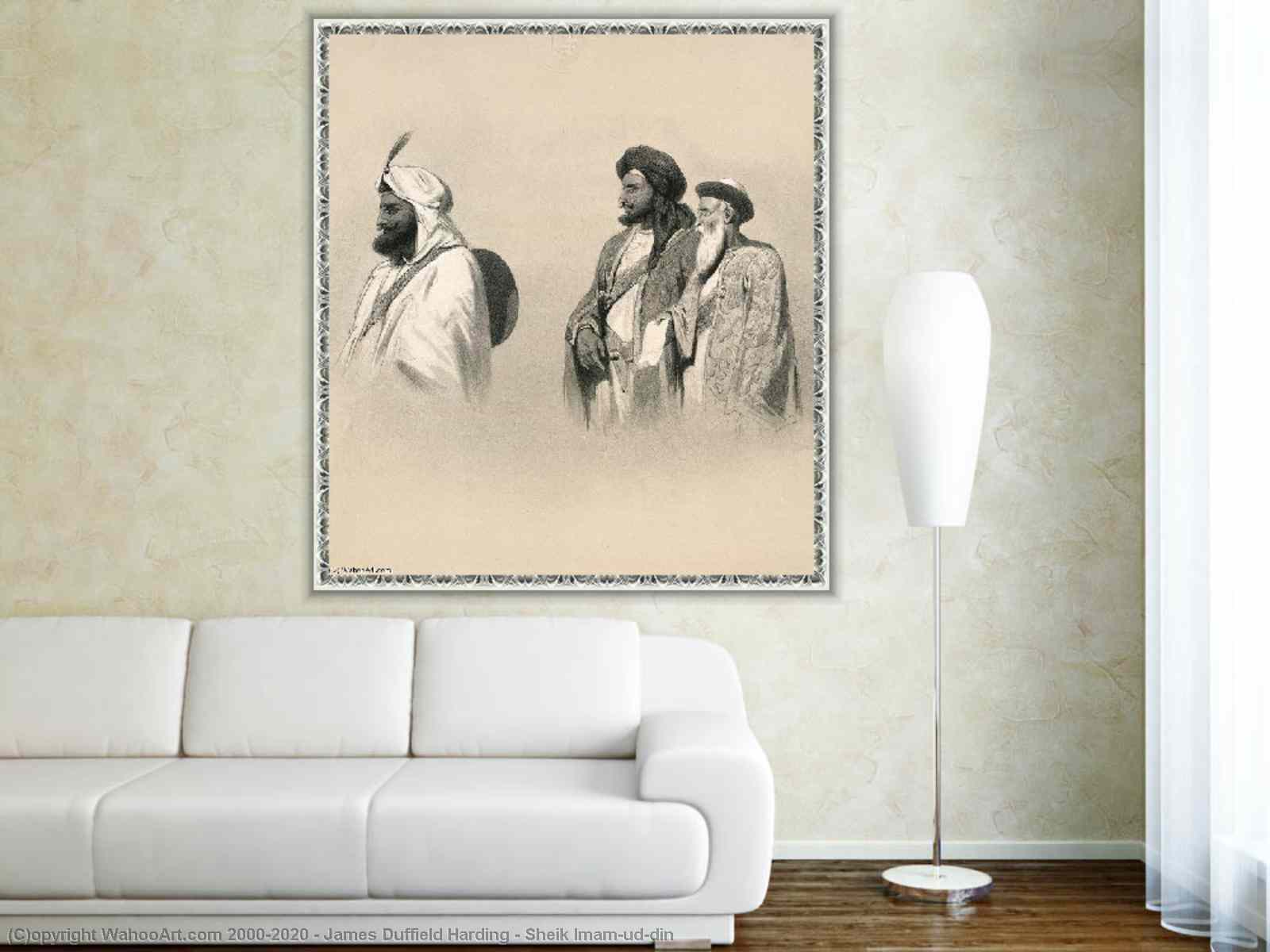The photograph captures a well-furnished living room featuring a sleek and modern white leather couch with low arms and no feet, situated on a dark, shiny hardwood floor. Adjacent to the couch, on its right, stands a contemporary and somewhat cylindrical lamp with a silver base and a bubble-like white lampshade, indicative of modern design. The room's wall showcases a sophisticated two-tone beige wallpaper with a subtle tan print, lending an elegant touch to the space. Dominating the wall is a large framed artwork with a white and black frame, portraying three Middle Eastern men. The man on the left is dressed in all white with a white turban adorned with a black feather and carrying a backpack; he also has a beard. In the middle stands another man wearing a colored turban and a well-tailored jacket. The man on the right, the eldest, has a white beard and wears a jacket and hat. The image also bears an artist's watermark at the bottom left corner, reading "Copyright Wahooart.com, 2002-2020 James Duffield Harding Sheikh Imam Ud-Din." To the far right, a long, transparent linen curtain frames a window, adding a touch of softness to the room's aesthetic.